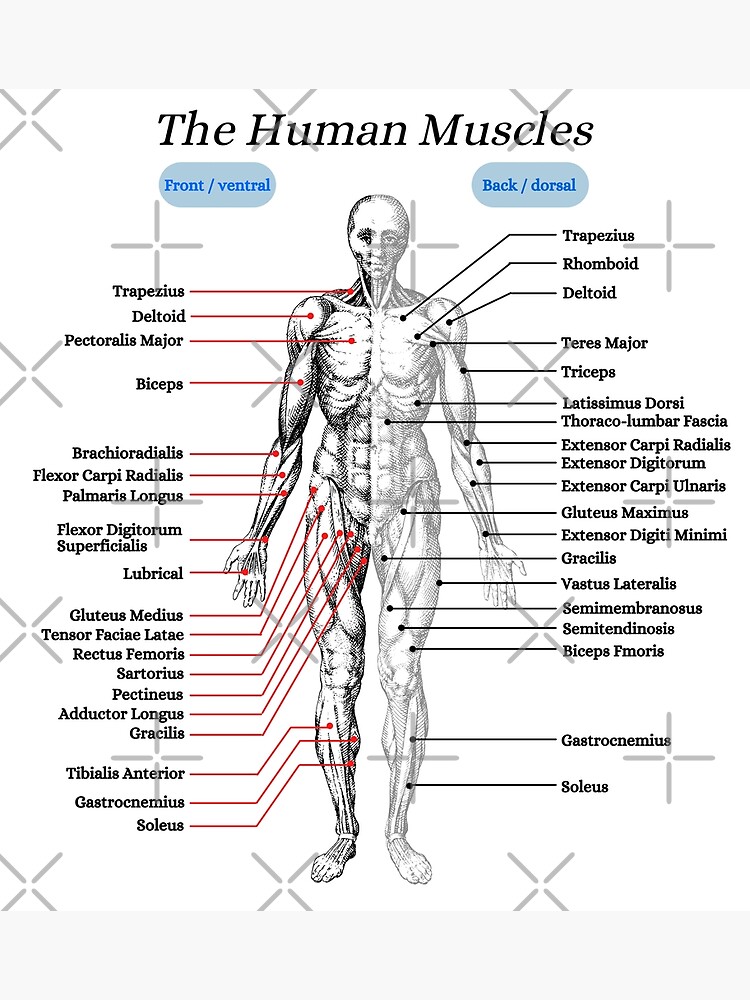This detailed educational illustration of the human body muscles, designed likely for a biology class, features both front (ventral) and back (dorsal) views. The top of the diagram has the title "The Human Muscles" in bold black letters with "T," "H," and "M" capitalized. The background has a white and gray rectangular shape with a pattern of X's and plus signs. The ventral view on the left and dorsal view on the right are split by a vertical divide. Each muscle group, such as the biceps, triceps, pectoralis major, trapezius, deltoid, soleus, and many others, is labeled with lines pointing from the muscle to its name. Additional labeled muscles include brachioradialis, flexor carpi radialis, palmaris longus, gluteus medius, tibialis anterior, gastrocnemius, latissimus dorsi, thoracolumbar fascia, gluteus maximus, semimembranosus, and biceps femoris, among others. The lines and labels make it a highly informative and visually comprehensive tool for learning the complex muscle structures of the human body.